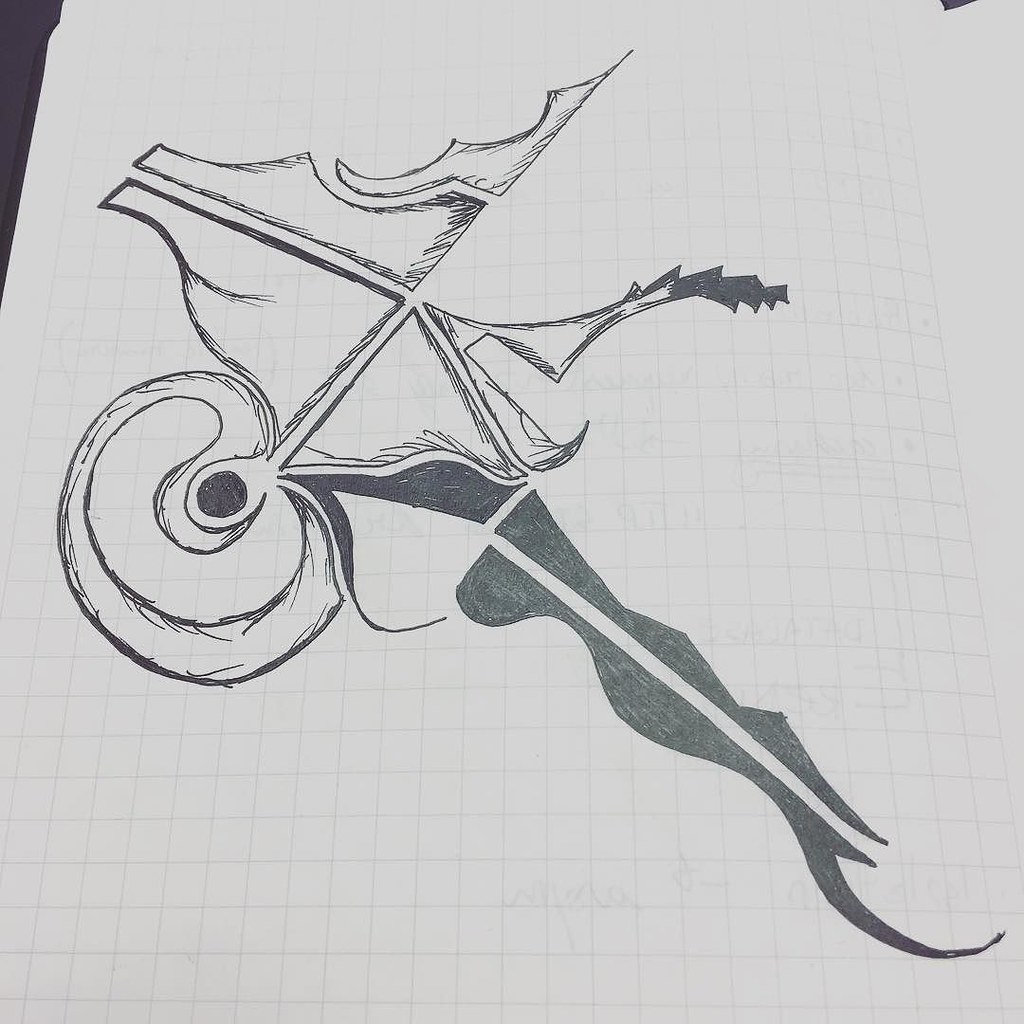This intricately detailed drawing is set on a sheet of faintly grid-lined paper, providing a subtle geometric backdrop to the artwork. The composition features bold line work that initially forms a pretzel-like semicircle, looping elegantly back into itself. The design evolves as it extends upwards and branches into three distinct segments, reminiscent of the sails on a sailboat, tilted slightly towards the left. On the right side, the shape transitions into a triangular form, accentuated by two wavy lines trailing off in a dark gray hue. This section evokes the impression of flames or flowing elements, adding a dynamic sense of movement to the abstract figure. The overall style is ornate and complex, blending abstract elements with a cohesive, artistic flow.